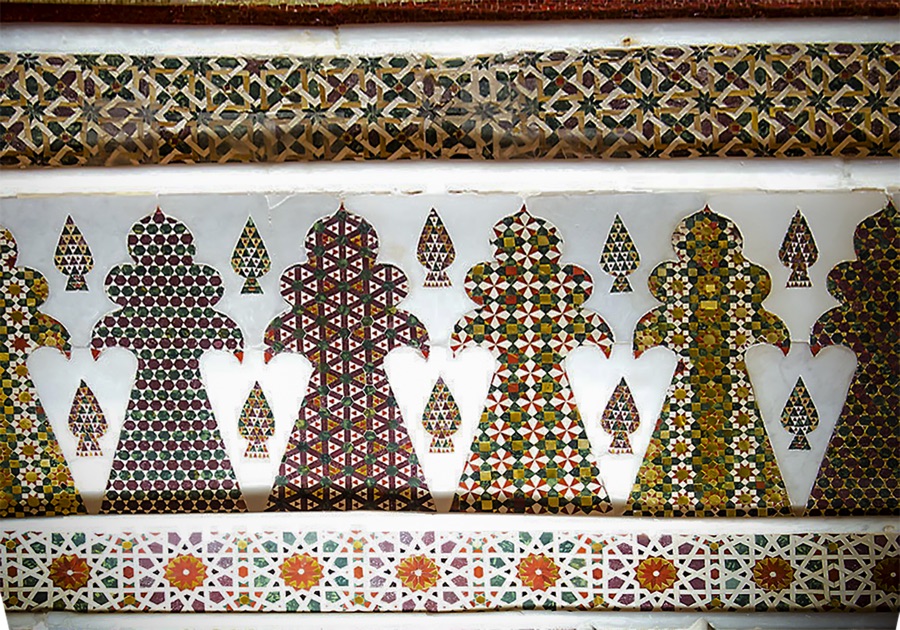The image showcases a decorative mosaic pattern, likely situated on a building wall. The design features a series of six repetitive shapes resembling trees or possibly silhouettes of princesses or witches, intricately adorned with smaller mosaic tiles in a variety of shapes, including rectangles, pentagons, and hexagons. These larger tree-like structures alternate with smaller, similarly shaped motifs, creating a visually appealing repetitive pattern. The color palette is rich and diverse, incorporating shades of brown, red, orange, green, maroon, gold, and white. Two prominent bands, one at the top and one at the bottom, frame the mosaic with repeated designs. The top part of the mosaic appears older and more simplistic, while the middle segment, dominated by beige and bright white bands, adds a vibrant contrast. The overall arrangement is intricate and colorful, resembling a carefully crafted artifact or a decorative element of architectural significance.